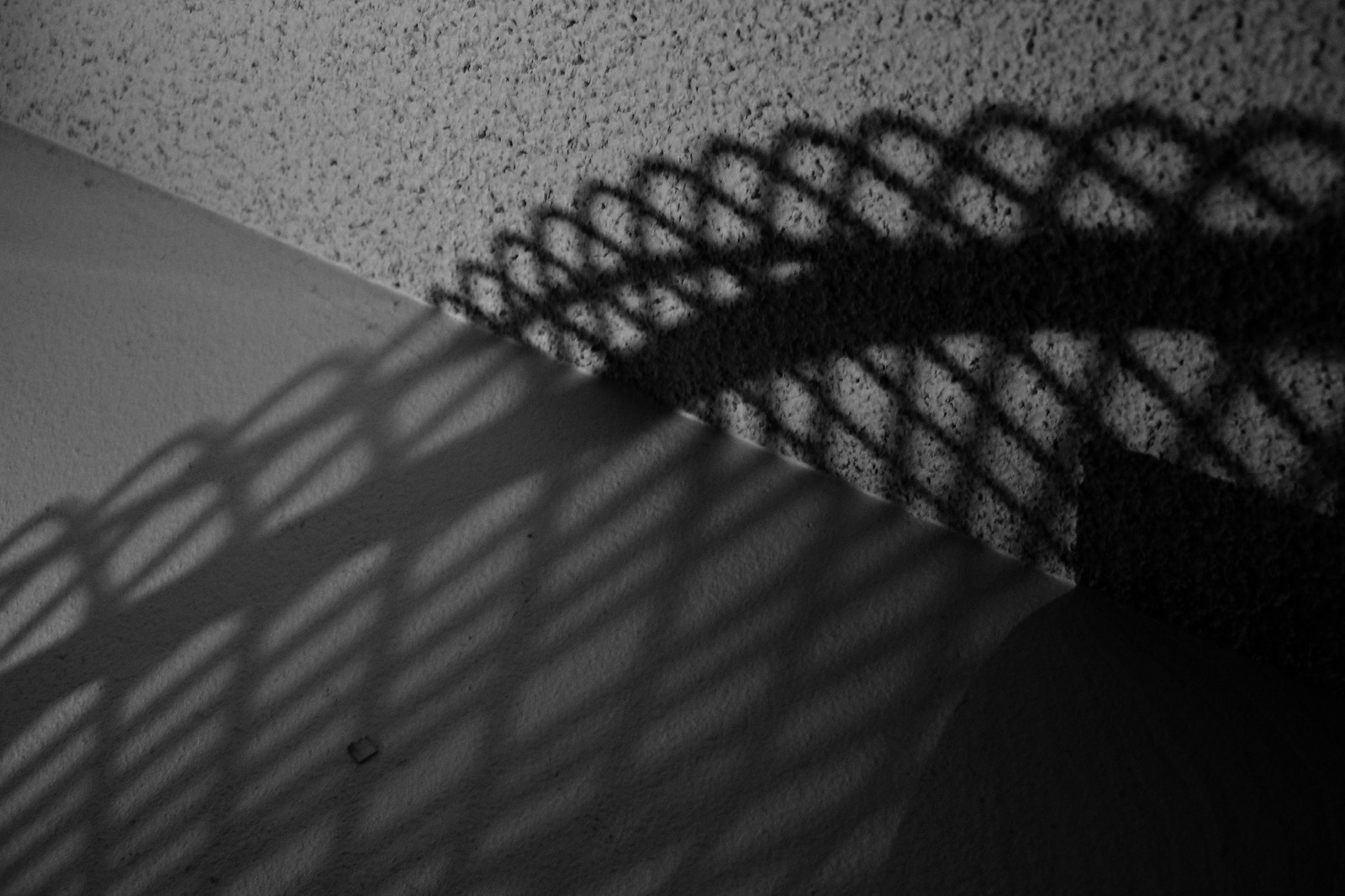This black and white photograph presents an abstract scene where a wall meets a concrete floor, creating a stark and shadowy corner. The image is shrouded in darkness, with only subtle textures visible—the traditional stucco finish on the wall and a layer of paint on the concrete floor. Dominating the composition is a shadow cast against the wall, possibly belonging to a wicker piece of furniture or some form of installation artwork. In the corner, a vague black shape can be seen, perhaps a silhouette of a vase or a cat, yet it remains indistinguishable due to the profound darkness. The image's obscurity and minimalistic elements evoke an artistic essence, showcasing the photographer's deliberate intention to capture an abstract, beautifully enigmatic moment.